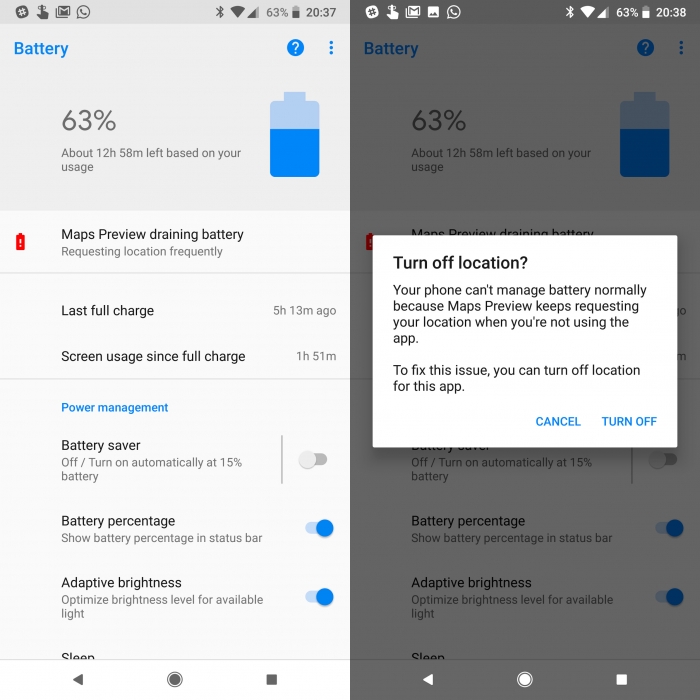The image collage displays two smartphone screens side-by-side, detailing battery usage statistics and suggestions for improving battery life. 

The smartphone on the left showcases the following information: Battery at 63% with an estimated 12 hours and 58 minutes of usage remaining at the current rate. It highlights that the "Map Preview" feature is excessively draining the battery by frequently requesting the device's location. Further details show that the last full charge was 9 hours and 13 minutes ago, with screen usage accounting for 1 hour and 51 minutes since that charge. It provides settings for power management, including a Battery Saver mode that activates automatically at 15%, the option to display battery percentage in the status bar, and Adaptive Brightness to optimize brightness based on available light.

The image on the right is a grayed-out version of the left screen, with a prominent pop-up box in the foreground. The pop-up reads: "Turn off location. Your phone can't manage battery normally because 'Map Preview' keeps requesting your location when you're not using the app. To fix this issue, you can turn off location for this app."